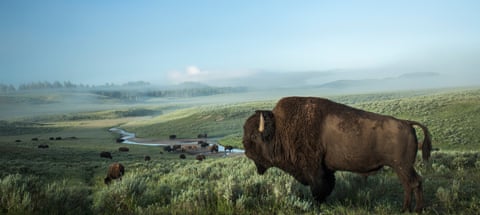In this captivating image, a prominent bison commands the foreground, occupying approximately a fourth of the total view while facing left. Its dark brown fur covers the head and muscular shoulders, tapering to sparser, shorter brown hair around its ribs and hindquarters. The bison stands amid knee-high green grass, surrounded by an expansive prairie. To the left and center in the background, a distant herd of bison speckles the landscape like dark brown spots, enhanced by the presence of a horizontally flowing stream. Extending further are lush green hills, blending seamlessly into a light blue sky, adorned with faint clouds and a hint of a white sun, casting a serene glow over the scene.